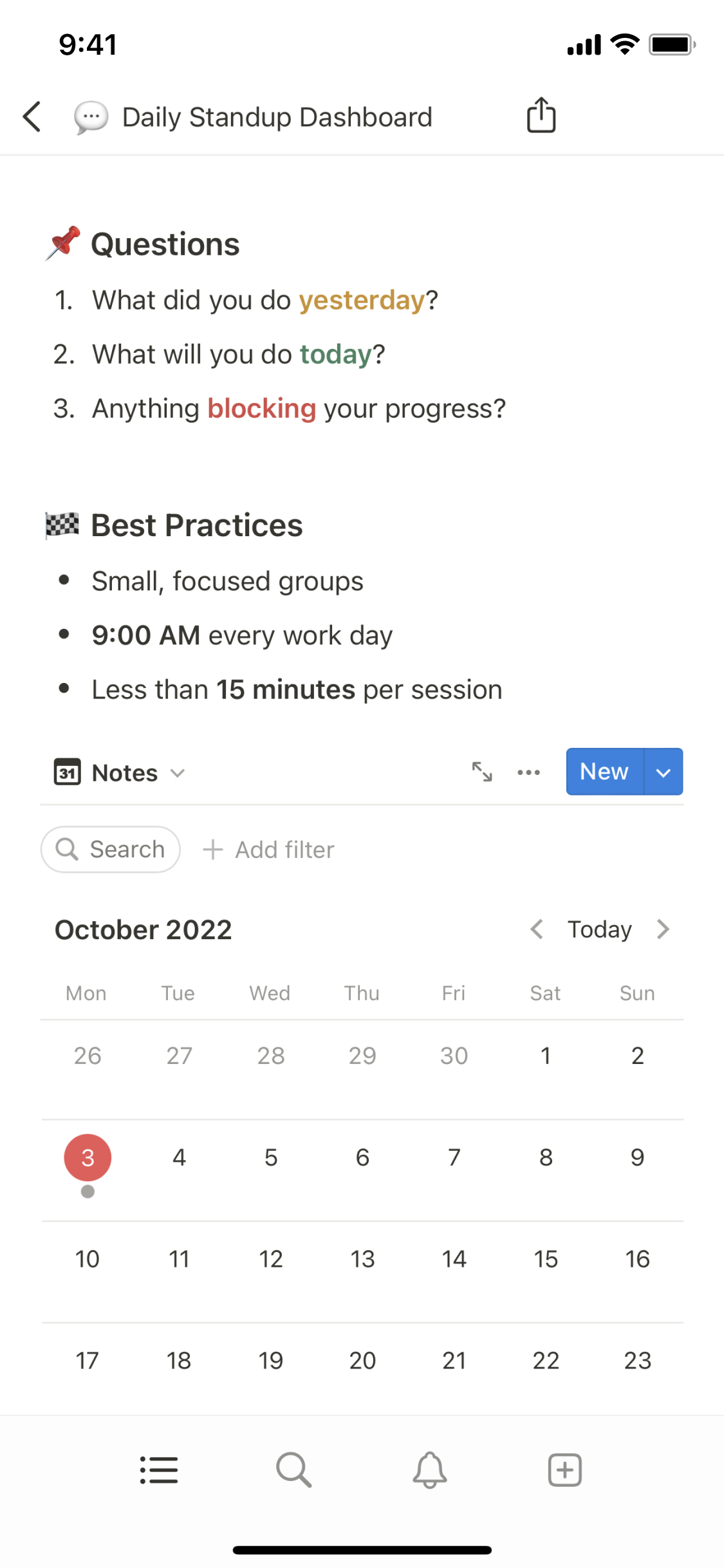In this particular screenshot, the background is entirely white with all text written in black, providing a stark and clear visual contrast. It is marked with a timestamp of 9:41 AM at the top. Below the timestamp, a series of questions are presented in black text interspersed with color-coded highlights and icons for emphasis:

1. "What did you do yesterday?" - Accompanied by a small pen icon and the word "Yesterday" highlighted in yellow.

2. "What did you do today?" - The word "Today" is emphasized in green.

3. "Anything blocking you from progress?" - This question appears without any additional color highlights.

Following these questions is a section labeled "Best Practices." This segment details recommendations for conducting focused group meetings: "Small focus groups, 9 o'clock AM every workday, less than 15 minutes per session."

Below this section is an area designated for notes, featuring a prominent, blue-colored "New" button, signifying where new notes can be added. The page also includes a calendar for the month of October, with October 3rd specifically highlighted, possibly indicating the current or a significant date.